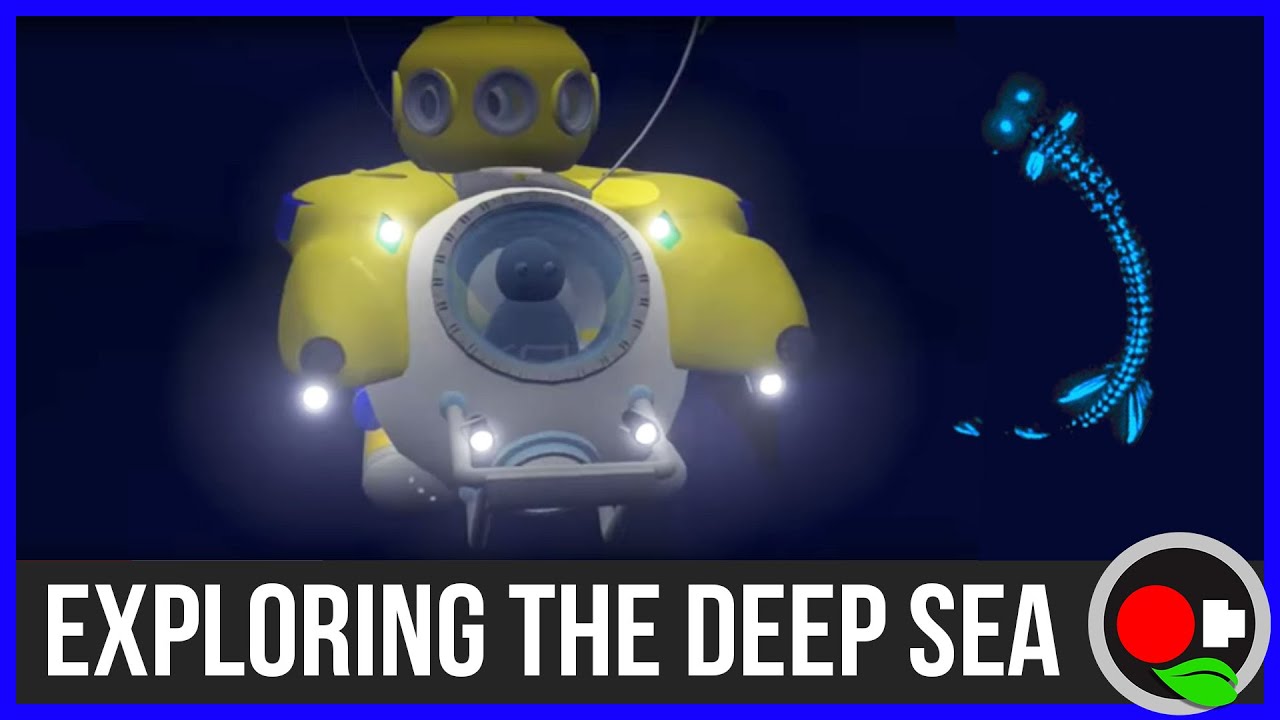A vividly detailed illustration showcases an undersea exploration robot prominently set against a black background, occupying most of the left side of the image. The robot itself is predominantly yellow, with a central gray section featuring a clear window that reveals a simplistic black figure, akin to a person, peering out. This windowed area is encircled by multiple bright lights: two on each side of the yellow exterior and two acting as headlights on the gray section. The robot's head has a greenish-yellow hue with numerous circular windows encircling it, suggesting a high-tech design.

Below the robot, a gray banner displays the phrase "Exploring the Deep Sea" in white lettering, emphasizing the image's theme. To the right of the text, there's a distinctive emblem comprising a red circle, a green leaf, and a white sideways T, adding an element of mystery and exploration. Additionally, an illuminated eel-like creature appears to the side, completing the underwater scene. Above the emblem, some tubing is visible, hinting at the robot's operational mechanics. The visual style of the illustration resembles early computer animations, evoking a sense of nostalgia and adventure.